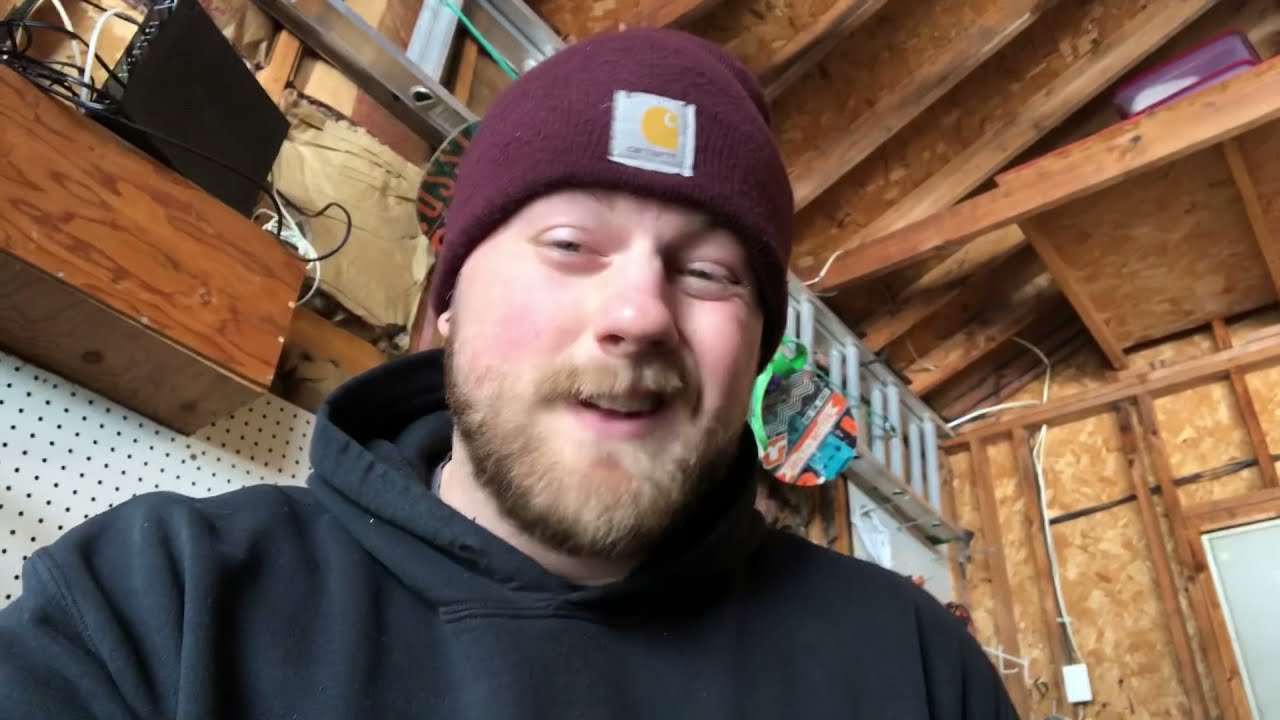The image depicts a younger to middle-aged white man situated slightly to the left of center frame within what appears to be an unfinished garage or shed. The man, who has pale skin and a reddish-brown beard, dons a black hoodie and a maroon Carhartt beanie with a white label. His facial expression shows a squinty-eyed look with a half grin that's more pronounced on the left side of his mouth. The setting around him is characterized by exposed wooden beams in the ceiling and uninsulated walls. Notable items in the background include a large extension ladder attached horizontally near the ceiling, a pegboard for hanging tools behind his left shoulder, some homemade shelving, and possibly a chainsaw or leveler. The overall scene suggests an environment in the process of construction or used as a workspace.